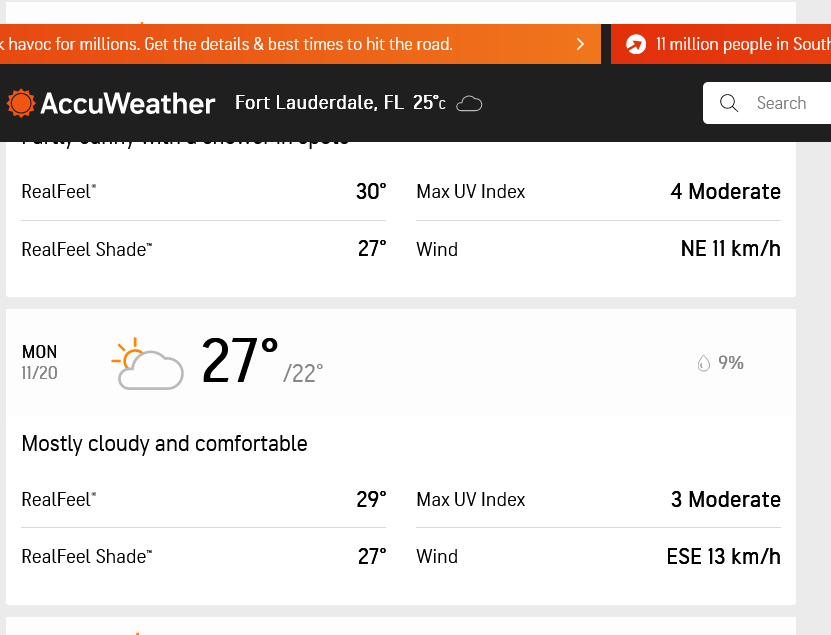This image captures a page from the AccuWeather website, illustrating a detailed weather forecast and layout. At the top of the webpage, there is an orange banner divided by a thin black line, followed by a red border. The orange banner features the text, "Havoc for millions, get the details and best times to hit the road," with an adjacent right-facing arrow leading into the black line. The red border contains another right-facing arrow and a white circle, hinting at impacts on millions in the south.

Beneath these colorful banners lies a black border housing the AccuWeather logo, comprising a sun icon and the word "AccuWeather." Positioned to the right of this logo are the details for Fort Lauderdale, Florida, showing a temperature of 25 degrees Celsius with a cloud icon, followed by a search box.

The main body of the webpage is white, detailing various weather metrics. It states a "RealFeel" temperature of 30 degrees Celsius, with "Max UV Index: 4 (Moderate)" to its right. Directly below, it lists a "RealFeel Shade" temperature of 27 degrees Celsius and a wind speed and direction of "Northeast, 11 km/h."

Additionally, forecast details for Monday, November 20th are provided: "Partly sunny" with a corresponding weather icon, a high of 27 degrees Celsius, and a low of 22 degrees Celsius. Further to the right, it indicates a 9% chance of rain and a description of "mostly cloudy and comfortable." Further highlights include another "RealFeel" temperature of 29 degrees Celsius, a "Max UV Index" of 3 (Moderate)," and similar metrics like the "RealFeel Shade" temperature of 27 degrees Celsius and wind from the "East Southeast at 13 km/h."

The layout and detailed weather information aim to provide users with a comprehensive understanding of the current and upcoming weather conditions.